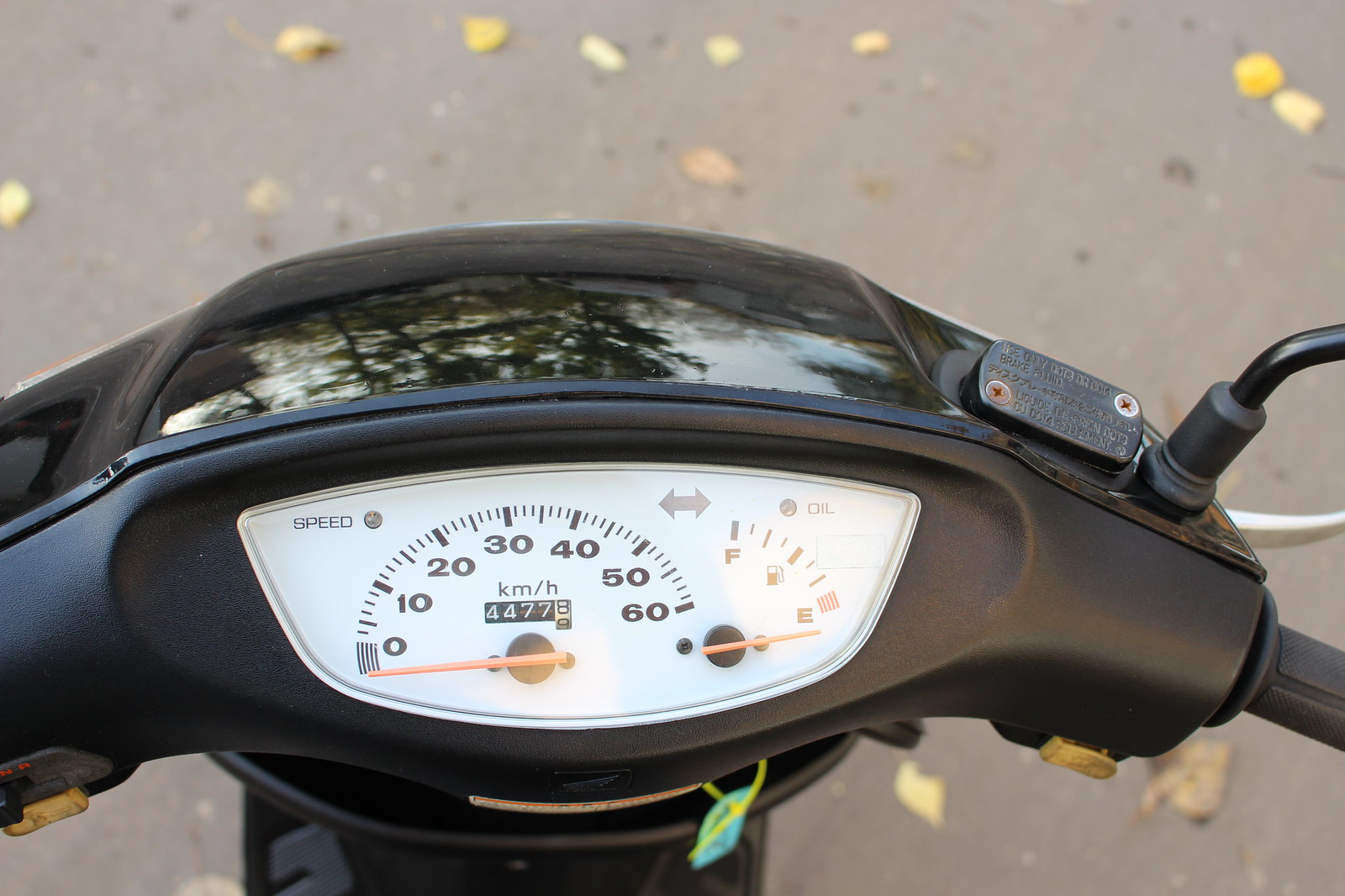An outdoor color photograph taken in bright daylight focuses on the dashboard of a moped-style motor scooter. The dashboard, positioned centrally, is somewhat oval in shape and features a white background. Prominently displayed is a semicircular speedometer ranging from 0 to 60, with major gradients marked at intervals of 10, 20, 30, 40, and 50. Minor hash marks are interspersed between the major gradients. Below the speedometer, the odometer reads 44.77 miles and an eighth of a mile in white letters. To the right of the speedometer is the fuel gauge, with its needle pointing horizontally to the far left, indicating the motorcycle is off. No lights or indicators are illuminated on the dashboard, suggesting the vehicle is parked.

The area above the speedometer, known as the cowl, is black. Visible is a portion of the right control handle and the stem that holds the right rearview mirror. The background at the top of the photograph shows a blurred surface of macadam with roughly 10 to 12 yellow leaves scattered, a subtle nod to the season. Similar leaves can be seen in the lower right background. Reflections of nearby trees are visible on the glossy black finish of the cowl, contrasting with the matte finish of the bezel surrounding the speedometer and fuel gauge.